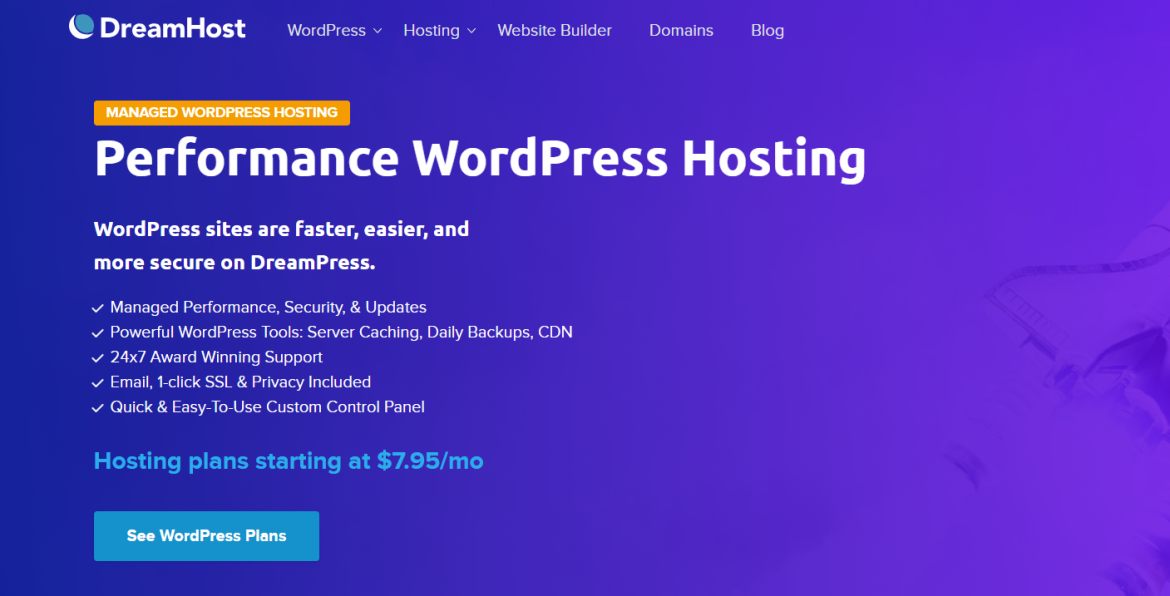In this detailed screenshot from the DreamHost website, we observe the interface highlighting their WordPress hosting services. The upper left corner prominently features the DreamHost logo. The main navigation bar offers various tabs labeled from left to right: WordPress, Hosting, Website Builder, Domains, and Blog. 

The central theme of the page is WordPress-related hosting services. The headline reads: "Managed WordPress Hosting" and "Performance WordPress Hosting." Below this, there’s a subheading that states, "WordPress sites are faster, easier, and more secure on DreamPress."

Several features are listed, emphasizing the service benefits: "Managed Performance, Security, and Updates," "Powerful WordPress Tools," "Server Caching," "Daily Backup," "CDN," "24x7 Award Winning Support," "Email," "One-Click SSL," and "Privacy Included." Another section highlights the ease of use: "Quick and Easy to Use" and "Custom Control Panel."

A call-to-action encourages users to explore further, with text stating, "Hosting plans starting at $7.95 a month," next to a prominent blue rectangle button with white text that reads "See WordPress Plans."

The website’s aesthetic features a sophisticated blend of purple and dark blue hues in the background, creating a visually appealing and professional look.